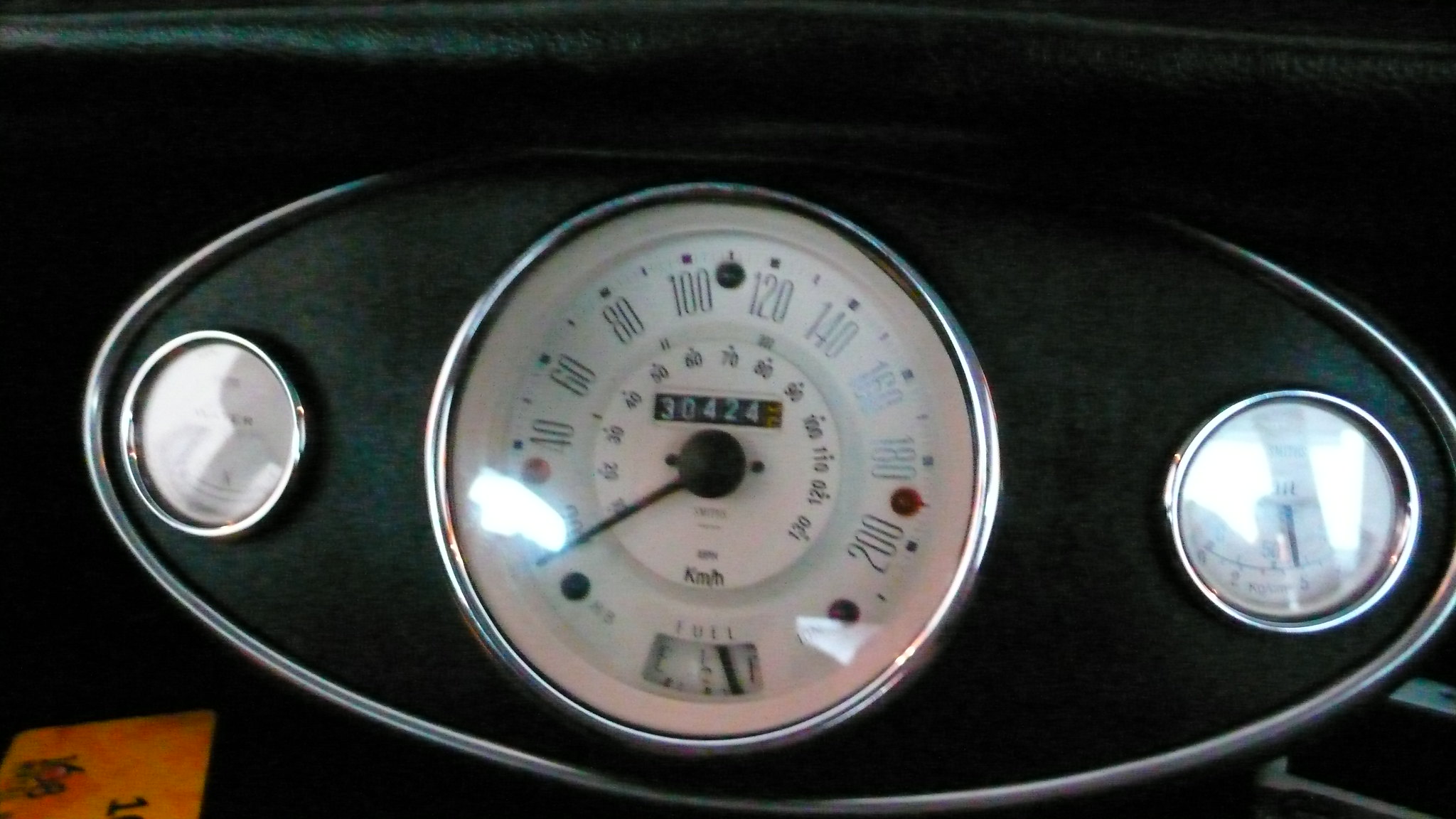The image depicts a vintage odometer with an oval shape, likely from a classic car. The device, which tracks speed and mileage, features a chromed outline adding a touch of elegance and age. It contains three displays: the central one for speed and two smaller circles on either side, all framed in chrome. The main speedometer, with a white background and black numerals, displays speed increments ranging from 0 to 200 mph, currently indicating 0 mph. The odometer shows a total mileage of 30,424 miles. The overall aesthetic hints at its historical value and classic design.